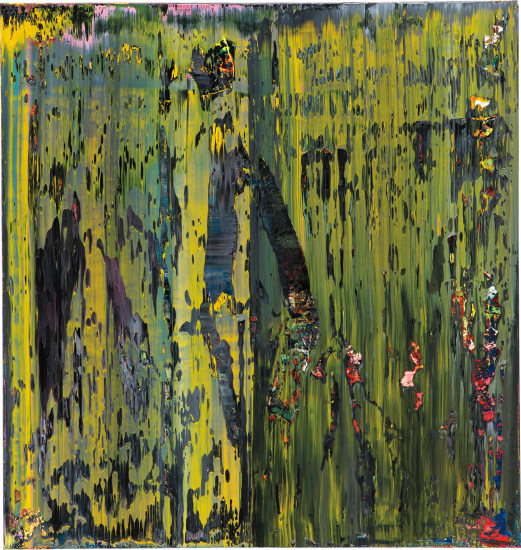The image depicts an abstract painting with a highly pixelated and blurry appearance. It features a diverse color palette dominated by various shades of green and yellow, interspersed with patches of black, gray, blue, and small speckles of red in the bottom right corner. The image is characterized by numerous vertical brush strokes that give it a modern and streaky look. There are no identifiable figures or objects within the artwork, enhancing its abstract nature. The artist appears to have applied multiple layers of paint, occasionally rubbing off parts to create a textured effect. Overall, it is a nuanced composition primarily conveyed through its energetic and fragmented use of color and form.